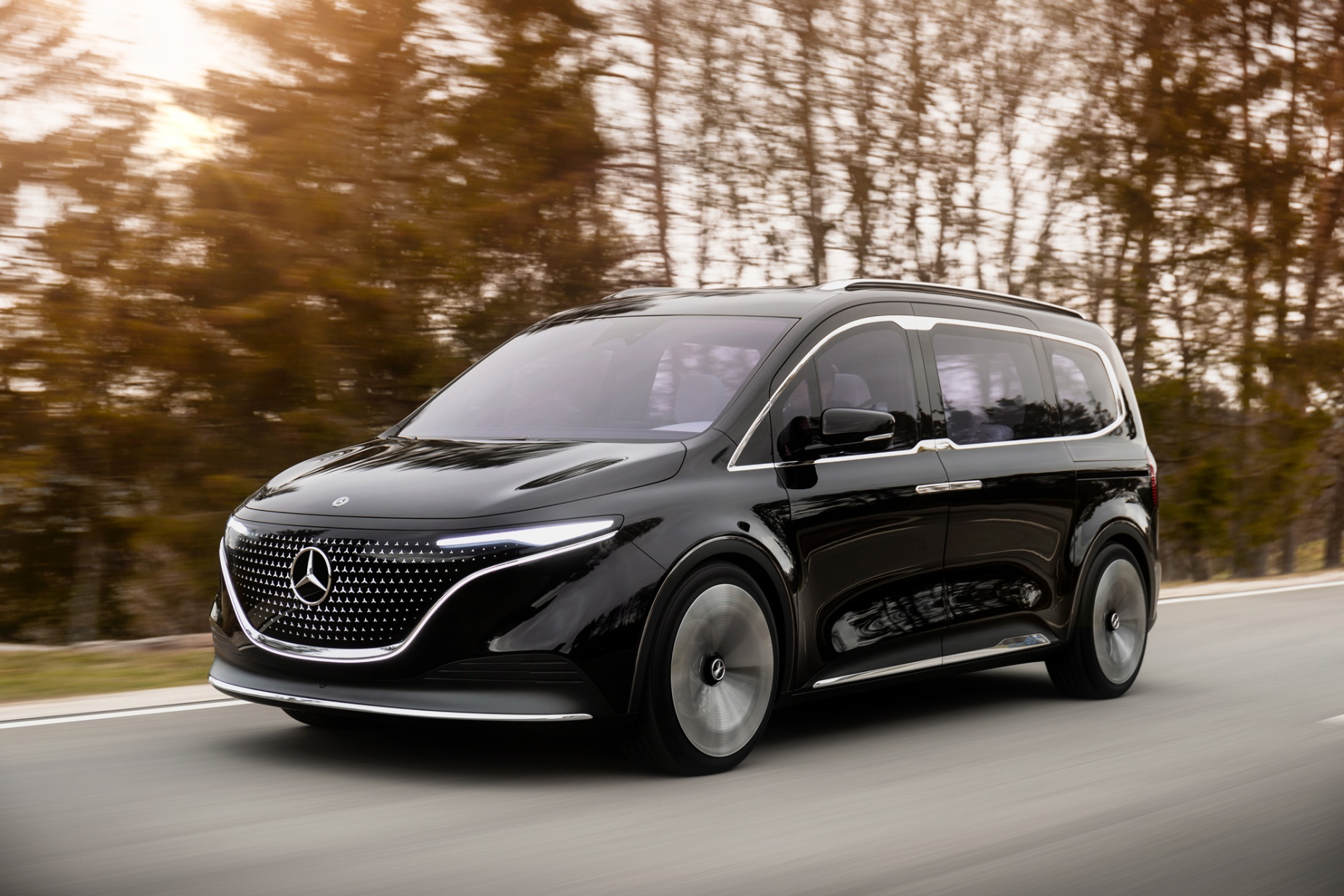The image captures a black Mercedes SUV in motion, driving swiftly down a road flanked by blurred, tall, skinny trees, indicating the vehicle's speed. The SUV features a sleek, modern design with a seamless front bumper, prominently displayed Mercedes emblem, and narrow LED headlights that enhance its sophisticated appearance. Reflections from the road's paint are visible on the car's side. The SUV is accented with chrome detailing around the windows and grille, and a roof rack is visible atop. Inside, a blonde woman is seen behind the wheel, with sunlight filtering through the treetops to the left, adding a dynamic and vibrant quality to the scene. The overall look is luxurious and contemporary, reminiscent of a high-end car advertisement aimed at modernizing the traditional minivan aesthetic into a more appealing and elegant form.